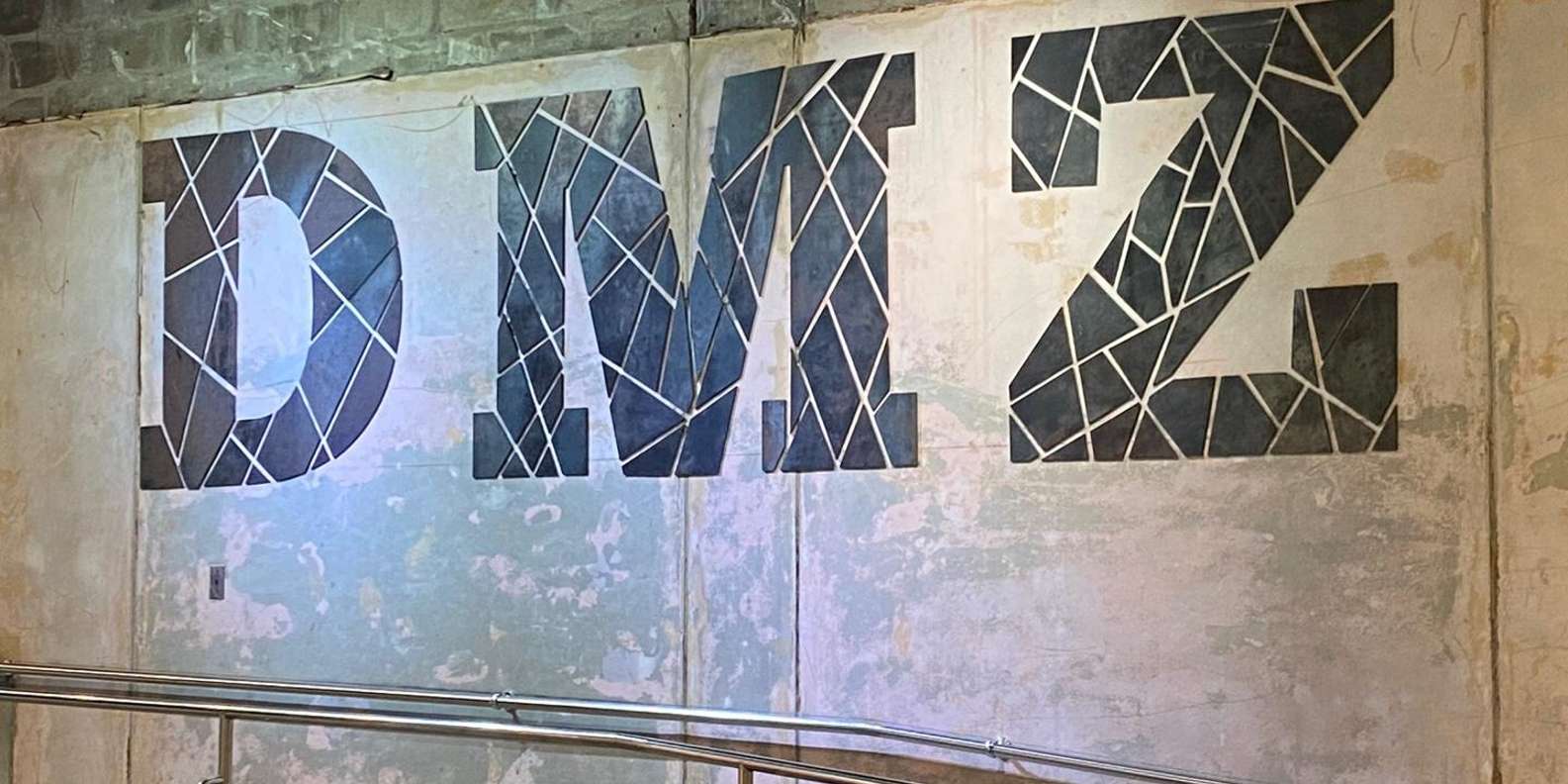In a dimly lit interior, the upper portion of an aged wall is made up of gray concrete blocks, fused together with visible mortar. The blocks bear the marks of time, showcasing various stains and discolorations. Below them, a series of panels have been affixed to the wall, originally a bright white but now faded and weathered. These panels interact intriguingly with the light, showing hues of light blue, peach, light brown, and gray amid the residual white. Adding an artistic touch, geometric shapes, predominantly black, though some appear blue due to the lighting, have been meticulously cut out and arranged to form the letters "D," "M," and "Z" across these panels. The composition creates a striking, albeit weathered, visual mosaic on this historical wall.